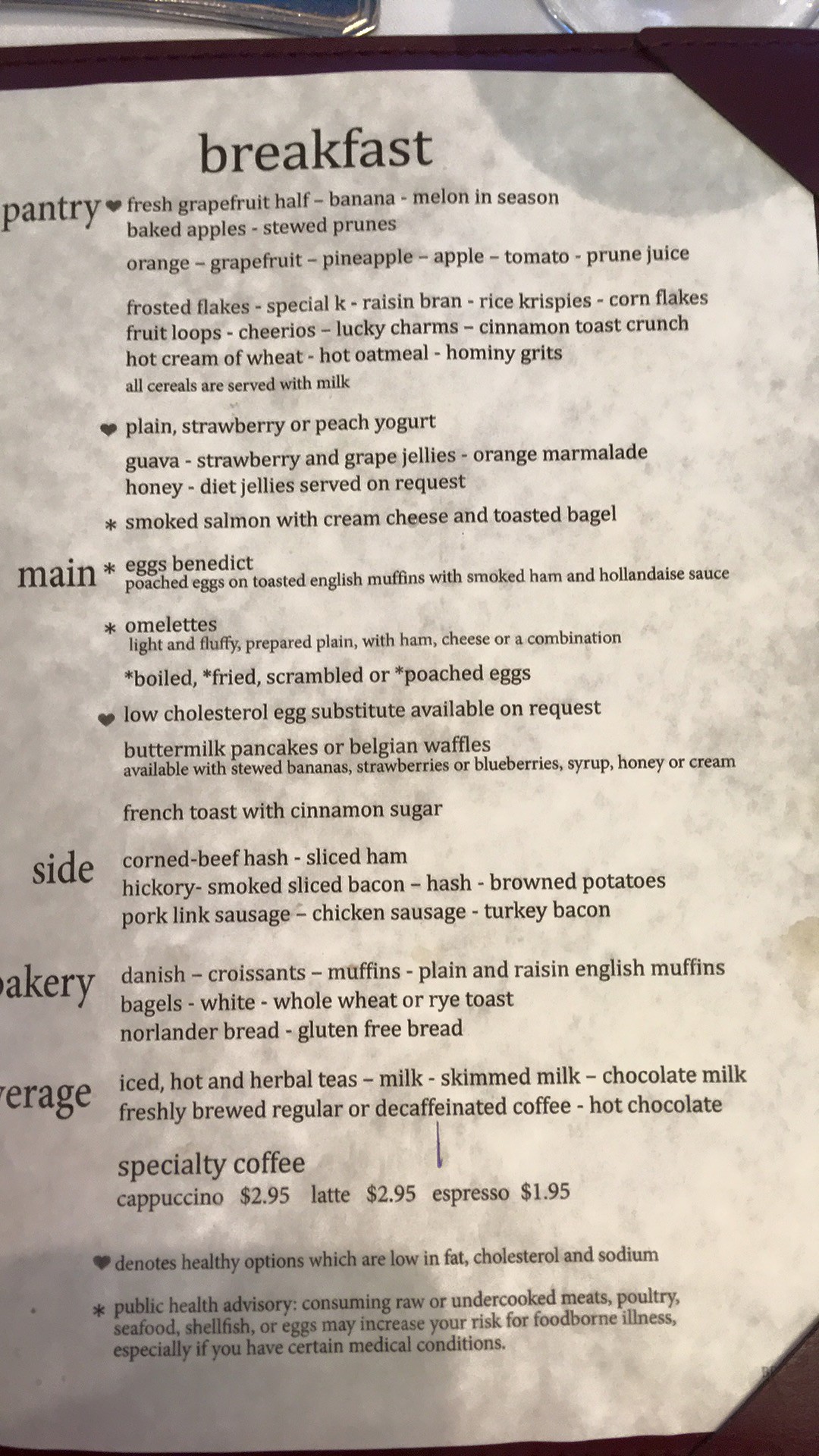A top-down photograph captures a breakfast menu in what appears to be a restaurant setting. The menu rests on a table that is likely draped with a white tablecloth, although the texture of the cloth is indeterminate. At the very top edge of the image, a narrow strip of the table is visible, running horizontally from left to right. Additionally, the top portion of the image shows the edge of a piece of silverware handle and the base of what looks like a wine glass.

The menu itself is printed on a paper with a very light beige hue, though it may appear this way due to the room's lighting. The paper features a mottled pattern with subtle gray tones. The word "breakfast" is displayed in lowercase letters at the top of the menu. Running down the left side of the page are main categories: "pantry," "main," "side," "bakery" (with the "B" partially cut off), and presumably "beverage" (with only "V" partially visible).

Beside these categories, descriptions list the available options. Under the "main" section, items such as "Eggs Benedict" and "omelets" are highlighted, along with a note mentioning a low-cholesterol egg substitute. The text of the menu is too extensive to detail in its entirety from this image.

The menu is encased within a deep purple folder, with its corners tucked neatly under the folder on the top right and bottom right of the image, adding a touch of elegance to the presentation.